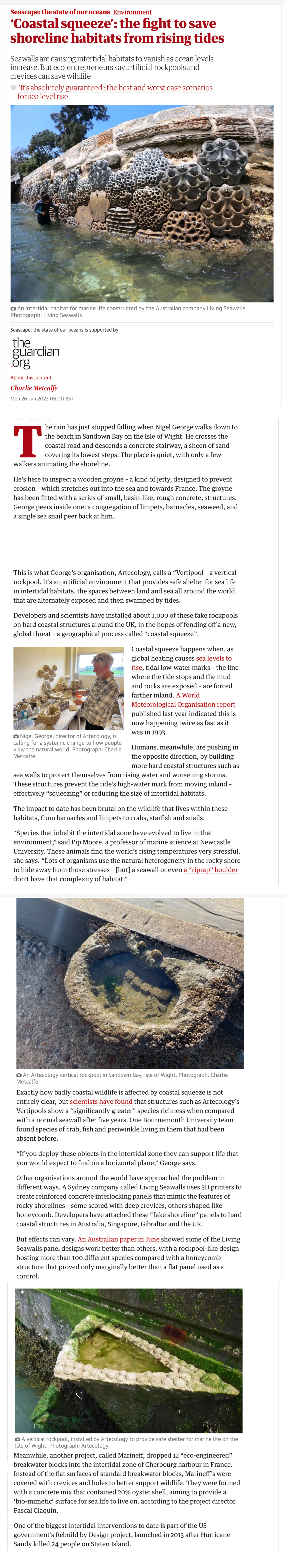The image is a long, narrow screenshot of an article titled "Coastal Squeeze: The Fight to Save Habitats from Rising Tides" in bold red text at the top. The text on the page is very small and difficult to read, with additional information in smaller black and red fonts. Below the title is an image showing a coastal scene with water, rocks, and possibly a beach. The article continues with small, unreadable black text interspersed with several small images. The first of these images appears near the top and is difficult to identify. Further down, there are pictures showing people and various scenes against rocks and greenery, which are also hard to discern due to their size. The smallest image is about halfway through the page, accompanied by some side text. The article is filled with text and a few more indecipherable images, including ones with triangular and circular shapes.